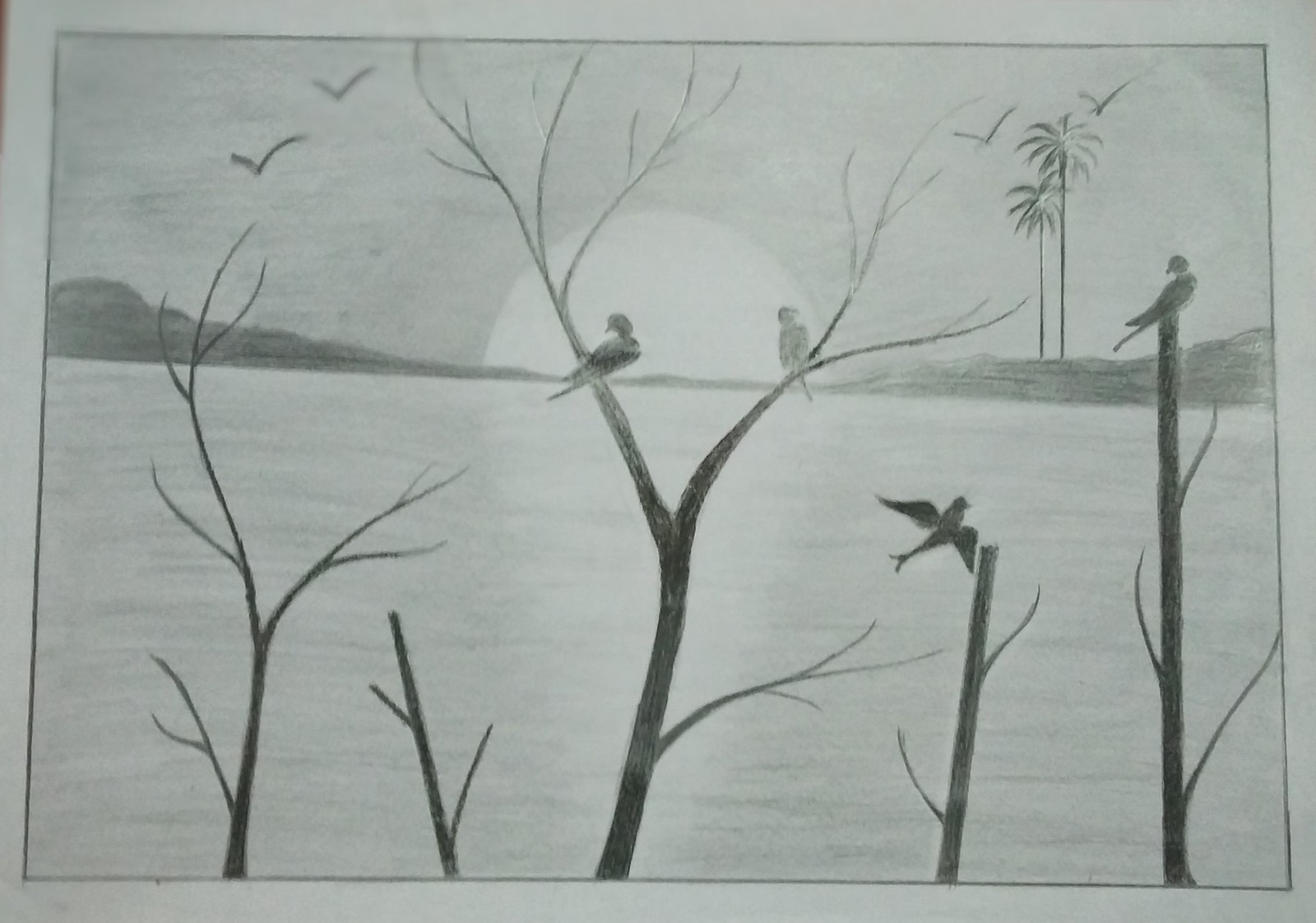In front of me is a meticulously crafted pencil drawing in black and white, presented on a light gray piece of paper with a defined black outline around the edges. The picture captures a serene sunset scene, where a perfectly rounded sun is either rising or setting over a calm, smooth body of water, subtly reflecting the light.

The foreground features five slender, bare trees with no leaves, their dark, shaded trunks and branches rising out of the water. Perched on these trees are several birds: two on the first tree, one on the middle fork of another, and another on a different branch, with a solitary bird preparing to land. Additionally, a couple of birds are flying through the sky, depicted with soft V-shaped formations to suggest movement.

Beyond these trees, on what appears to be a distant shoreline, there are tall, bushy palm trees and small hills or dunes. On one side of the horizon, a mountain silhouette can be made out, enhancing the depth of the landscape. The overall scene is delicate and tranquil, intricately combining nature's elements to create a captivating visual narrative.